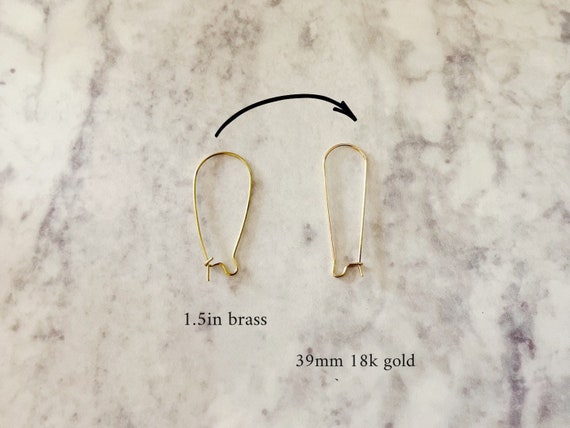This image presents a detailed comparison between two elongated clasps or hooks, positioned on a marble-like countertop that features a creamy white background with subtle bluish-grey and black veining. The clasp on the left is crafted from 1.5-inch brass and has a broad, tall design with a small catch at its base, reminiscent of a thickened earring hook. The counterpart on the right, fashioned from 39-millimeter 18-karat gold, stands slightly taller and slimmer, maintaining a similar shape but with a more refined and elegant profile. An annotation of a black arrow arches from the top of the brass clasp to the top of the gold clasp, drawing attention to the comparison between the two. Overall, the photograph highlights the distinct differences in material and dimensions between the brass and gold clasps while set against the muted, blurred elegance of the marble background.